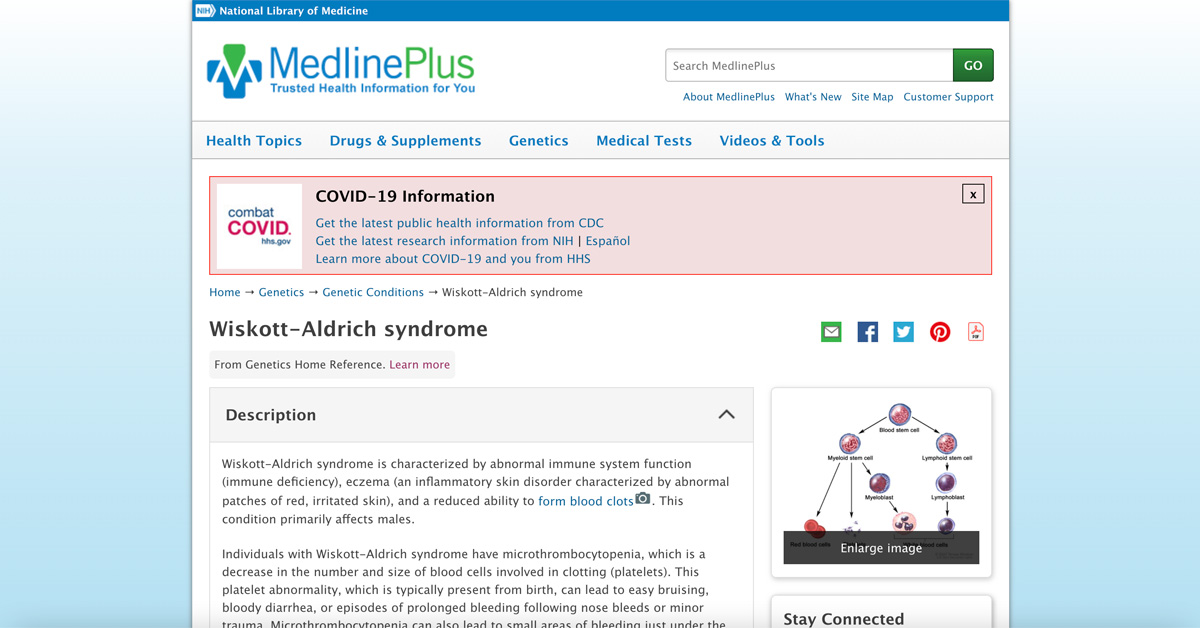The image from MedlinePlus features a dual white and blue border on both the left and right sides. At the top center, the webpage itself displays on a white background, with a prominent blue bar stretching across the top. The MedlinePlus logo appears here in green and blue, accompanied by a matching logo or symbol on the left. Directly below, the phrase "Trusted Health Information for You" is displayed, aligning with a search bar featuring a green "Go" button on the right.

Beneath the search bar, navigation tabs include "About MedlinePlus," "What's New," "Site Map," and "Customer Support." Further down, key health categories such as "Health Topics," "Drugs & Supplements," "Genetics," "Medical Tests," and "Videos & Tools" are listed. A highlighted section in red provides updated COVID-19 information. Below that, another spotlighted article titled "Wiskott-Aldrich Syndrome" appears.

The central content area includes a detailed description with several paragraphs, accompanied by images on the right. Additionally, social media links are available on the right side of the page.